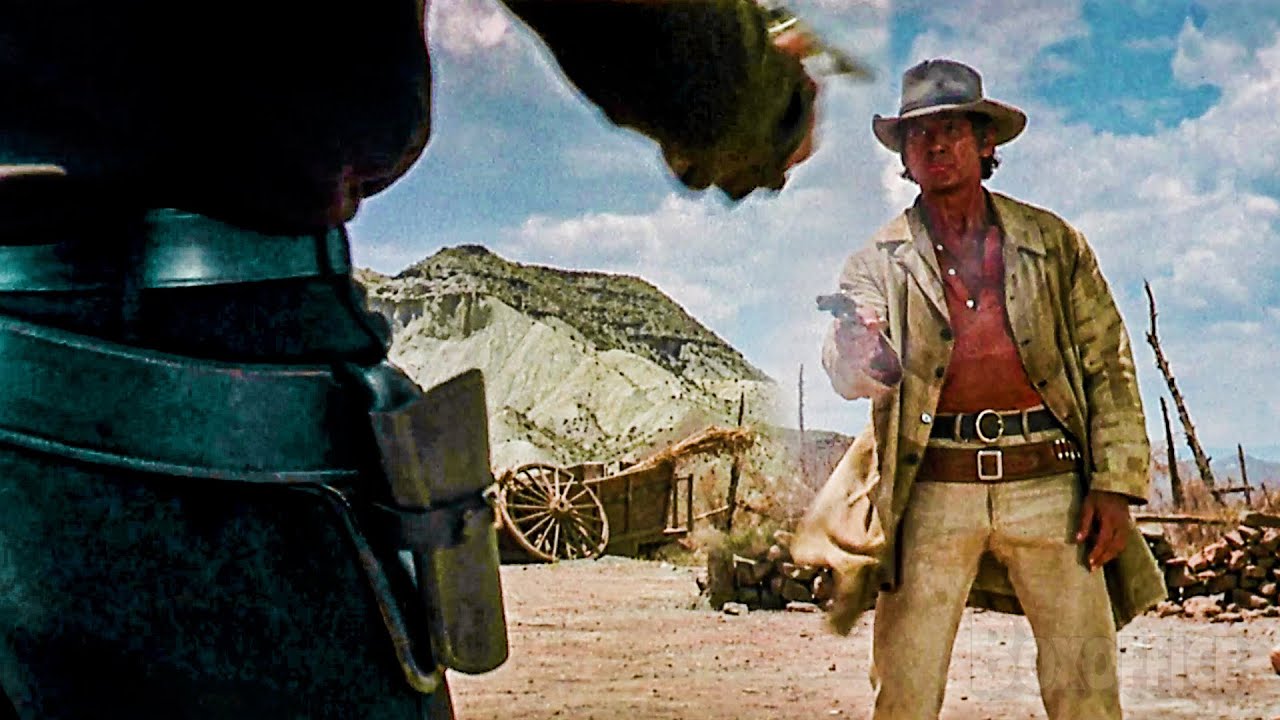The image is a still from what appears to be an old Western movie, potentially featuring Charles Bronson. The setting is outdoors with a blue sky dotted with puffy white clouds, and a mountainous backdrop partially visible through the grain. The ground is dusty and sandy, with a wagon wheel and broken wagon adding to the desolate, desert-like atmosphere.

The scene depicts a tense standoff between two gunfighters. The man on the right, likely the focal character, stands in a faded, possibly dirty, tan or cream-colored jacket and matching pants. He wears a gray or dirty cowboy hat, an orange-red shirt with white buttons, and has a black belt plus a brown leather gun holster with a metal buckle. His right hand is extended, holding a gun with smoke indicating he has recently fired.

On the left, only part of the other gunfighter is visible from the hip down. This character is dressed in all black—a long-sleeve shirt, pants, and a loose-fitting holster belt. His right arm is extended as he aims his gun at the man on the right.

The background includes a dilapidated building, various bits of debris, a wagon wheel, and hints of greenery adding to the barren feel of the wild west setting. The image exudes a classic Western duel atmosphere, with a stark contrast between the two characters and their grim, dusty surroundings.